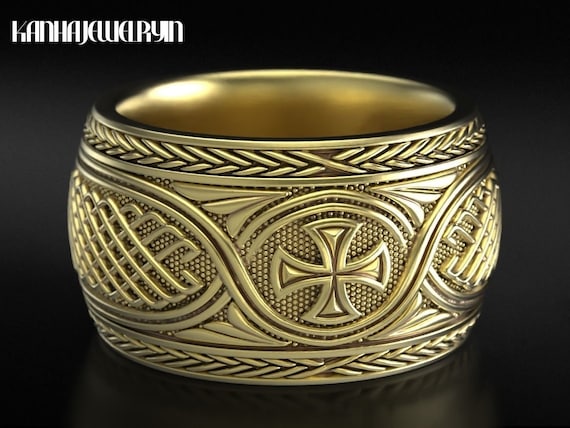This is an intricate and detailed gold ring, photographed in a way that it occupies the entirety of the frame against a black background, creating the illusion that it is floating in space. The lighting focuses on the ring, emphasizing its exquisite craftsmanship. The design features a central motif of Celtic knots intertwined with a delicate cross pattern, suggesting an ancient pre-Christian origin from the British Isles. Encircling this are woven wheat patterns, contributing to its Celtic style. Along the edges, there is a decorative criss-cross design with a helix-like shape in the middle. The interior of the ring is smooth, shining gold. In the top left-hand corner, white lettering reads "Canna Jewelry I.N.," presumably indicating the jeweler's name. The overall presentation highlights the ring's luminous gold color and its fine, intricate detailing.